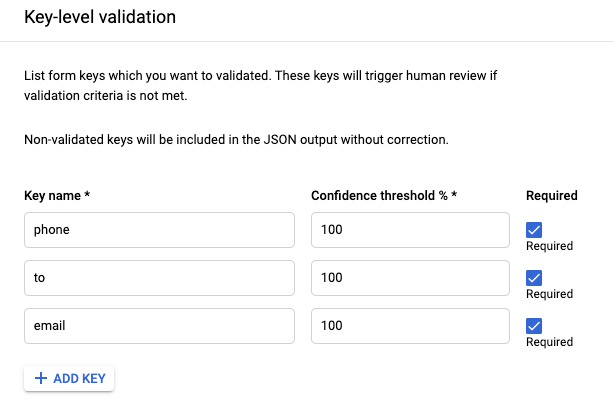In the image, there is a screenshot discussing key-level validation displayed on a white background with black text and distinct blue elements. At the top, the title reads "Key-Level Validation." Just below, a description explains: "List the form keys you want to validate. The keys will trigger human review if validation criteria are not met. The keys will be included in the JSON output without correction."

Beneath the description, a table is presented with three columns: "Key Name," "Confidence Threshold (%)," and "Required." The "Key Name" column lists three entries: "phone," "to," and "email." Corresponding to these keys, the "Confidence Threshold (%)" column indicates a value of "100" for each entry. In the "Required" column, each key is marked with a blue check box, indicating that they are required.

At the bottom left of the screenshot, a blue button labeled "Add Key" allows users to add additional key names to the table. The blue color is used solely for the "Add Key" button and the check boxes, contrasting with the otherwise black and white design.